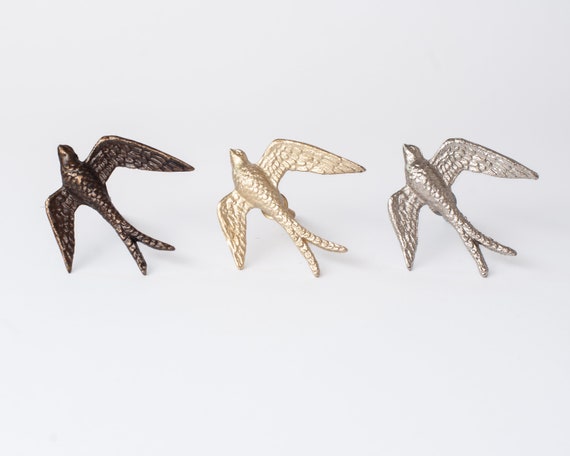This photograph showcases three intricately designed bird brooches set against a pristine white background. Each brooch features a bird with outstretched wings, captured mid-flight toward the top left corner of the image. The birds, which have detailed feather markings on their bodies and tails that split into two, resemble sparrows or doves. The bird on the left boasts a dark bronze color, the middle one is a pearly white with a light gold hue, and the bird on the right is a silvery pewter tone. All three possess a metallic sheen that appears to be painted rather than their natural material. Positioned diagonally, these brooches are seen from the underbelly, giving the sense that they are soaring with their beaks facing slightly upward, adding to the dynamic portrayal of flight. Shadows cast on the white surface enhance the lifelike quality of these elegant jewelry pieces.